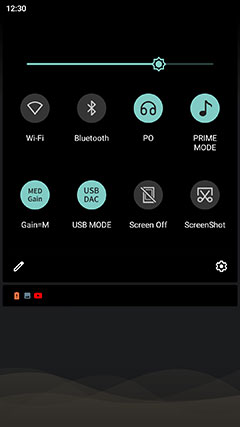This is a screenshot of a phone screen showcasing the pull-down menu. The menu features a gradient from light green to light teal at the top, with a circular slider designed to resemble the shape of a sun. Below this slider, there are two rows of circular icons and buttons. Some of these icons are gray, while others are light teal, each containing an icon or text with a label beneath it. 

The icons in the top row include:
- Wi-Fi 
- Bluetooth 
- PO 
- Prime Mode 

The icons in the bottom row are:
- Med Gain 
- USB Mode 
- Screen Off 
- Screen Shot 

The background of the menu is black, providing a sharp contrast to the icons. At the bottom of this section, there are two additional icons: a pencil icon on the left and a gear icon on the right, likely representing edit and settings functions respectively.